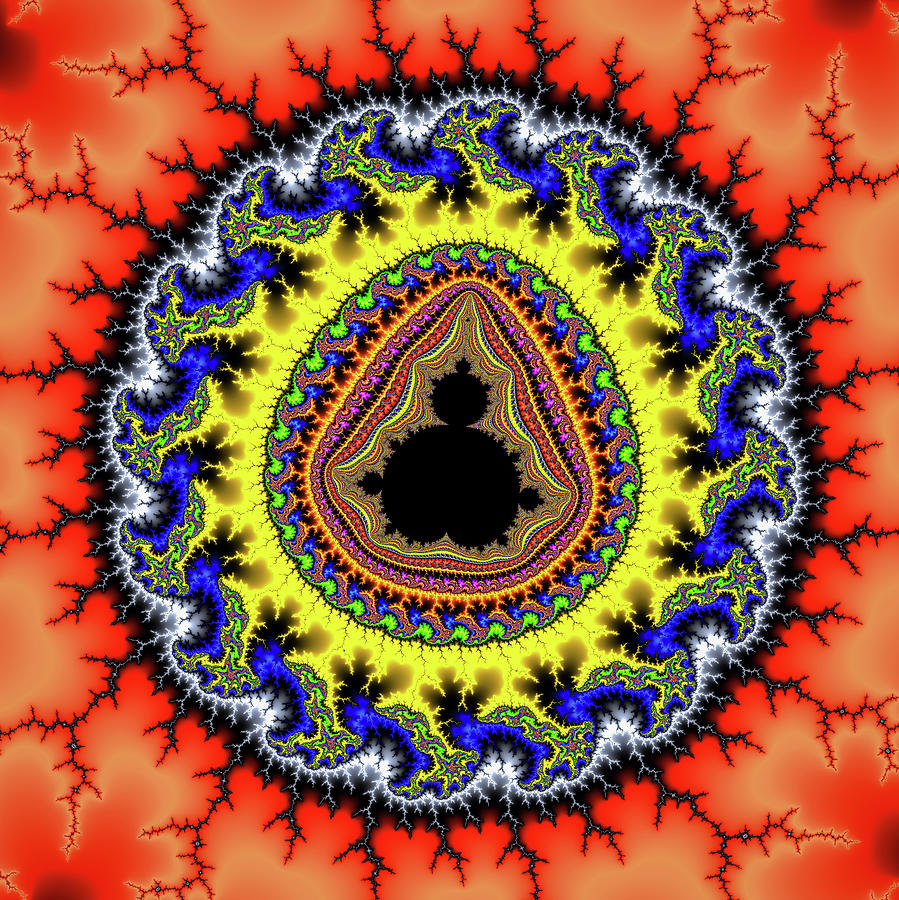This artistic piece is a vibrant, circular composition featuring a complex interplay of colors and patterns. The outermost layer depicts an intense red and orange gradient that evokes a sense of fiery energy, occasionally interrupted by streaks of blue, giving the appearance of flames or lightning strikes. Surrounding the center, multiple rings of colors emerge, including a prominent white circle, followed by sequences of blue, green, yellow, and pink, each interspersed with intricate patterns. The middle of the artwork, resembling an eyeball, is dominated by black, forming a central focal point that radiates outward. These color layers, almost wave-like, continue inward in a mesmerizing array of designs and shades, culminating in a deep black core with a smaller black circle just above it. The overall effect is a hypnotic and dynamic visual journey through diverse colors and textures.